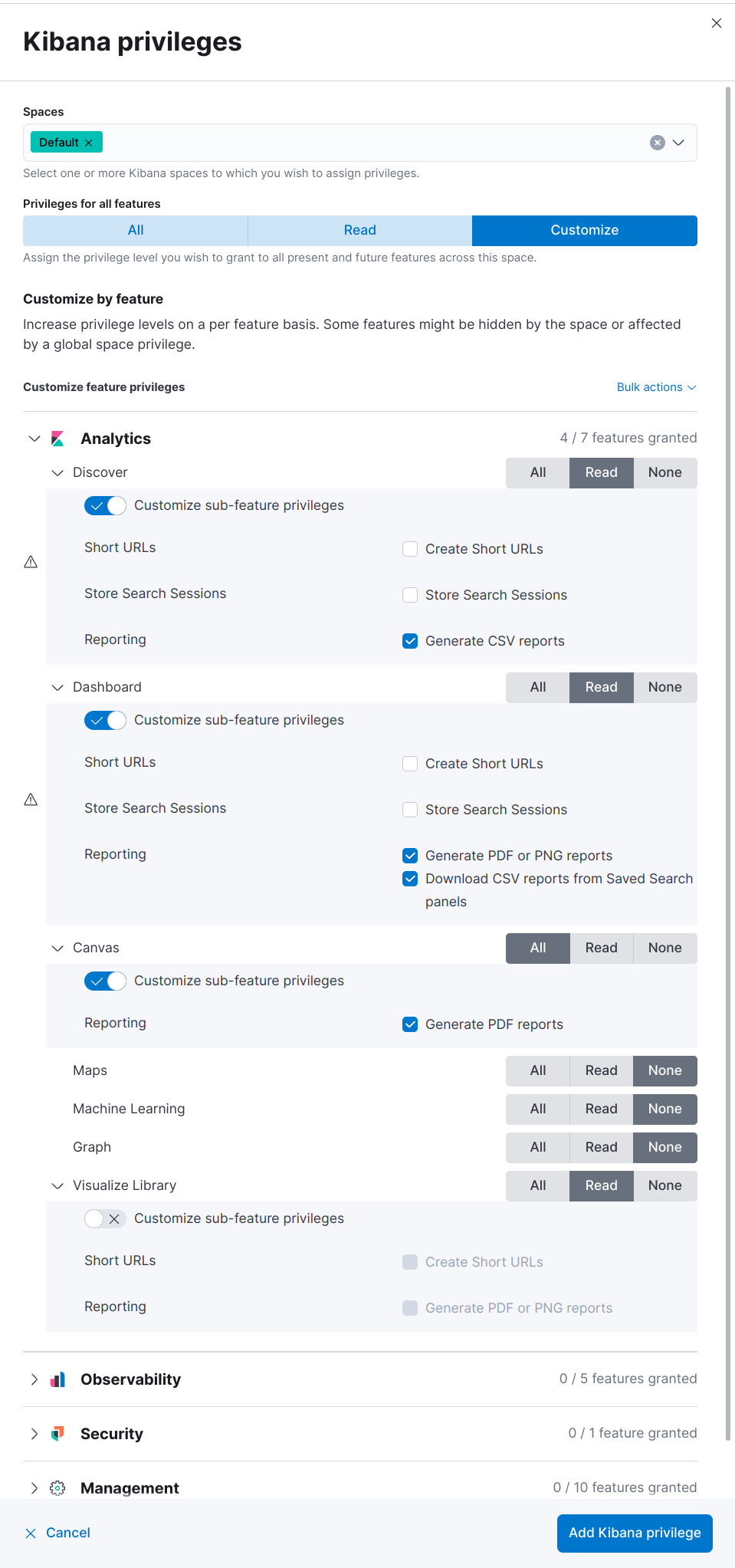This is a detailed screenshot illustrating the backend interface of Google Analytics, specifically focused on configuring Kibana privileges. The interface spans several sections, each delineated by thin gray lines and distinctively labeled.

At the top left corner, the title "Kibana Privileges" is prominently displayed in bold black lettering, providing clear context for the tasks being managed. On the top right corner, there is a small gray square, likely indicative of a minimized menu or auxiliary function.

The first section is labeled "Spaces," also in bold black text. Beneath this heading, a turquoise rectangle button with black text labeled "Default" is visible, suggesting a standard or primary configuration. An instructional line below advises: "Select one or more of Kibana spaces to which you wish to assign privileges." Further down, "Privileges for all features" is indicated in bold, and below that are three buttons for privilege settings: "All" and "Read" in sky blue rectangles, and "Customize" in a dark blue rectangle with white text.

Proceeding to "Customize by feature," bold black text introduces this next segment. Below, operational options for feature privileges are introduced, with a blue text "Bulk actions" accompanied by a down arrow on the right, indicating a dropdown menu.

The following section pertains to Google Analytics, starting with a recognizable Analytics logo on the left. Key features and configurations are listed downward on the left: "Discover," "Customize sub feature privileges," "Short URL," "Store search sessions," and "Reporting." In the upper right of this section, "4-7 features granted" is noted along with three horizontal gray buttons labeled "All," "Read," and "None."

Below, three privilege options for specific actions are presented with checkboxes: "Create short URL" and "Store search sessions" are unchecked, whereas "Generate CSV reports" has a blue checkbox indicating selection.

Further sections expand on specific areas like the "Dashboard," which highlights two selected privileges: "Generate PDF or PNG reports" and "Download CSV reports," both marked with blue checkmarks. Another section labeled "Canvas" shows similar configurations, with toggles for sub-feature privileges and options like "Generate PDF reports."

The brief "Customize sub feature privileges" section appears next in a gray shade, with a toggle button unselected and a gray "X" to its right. Detailed privileges for "Short URLs" and "Reporting" (including PDF and PNG report generation) are provided with unchecked gray checkboxes.

At the bottom, there are distinct sections for "Observability," "Security," and "Management," each marked by bold black headings and corresponding multicolored icons, with gray right arrows to their left. The interface concludes with action buttons: a "Cancel" button in blue on a gray background at the bottom left, and a blue rectangle labeled "Add Kibana Privilege" in white text on the bottom right.